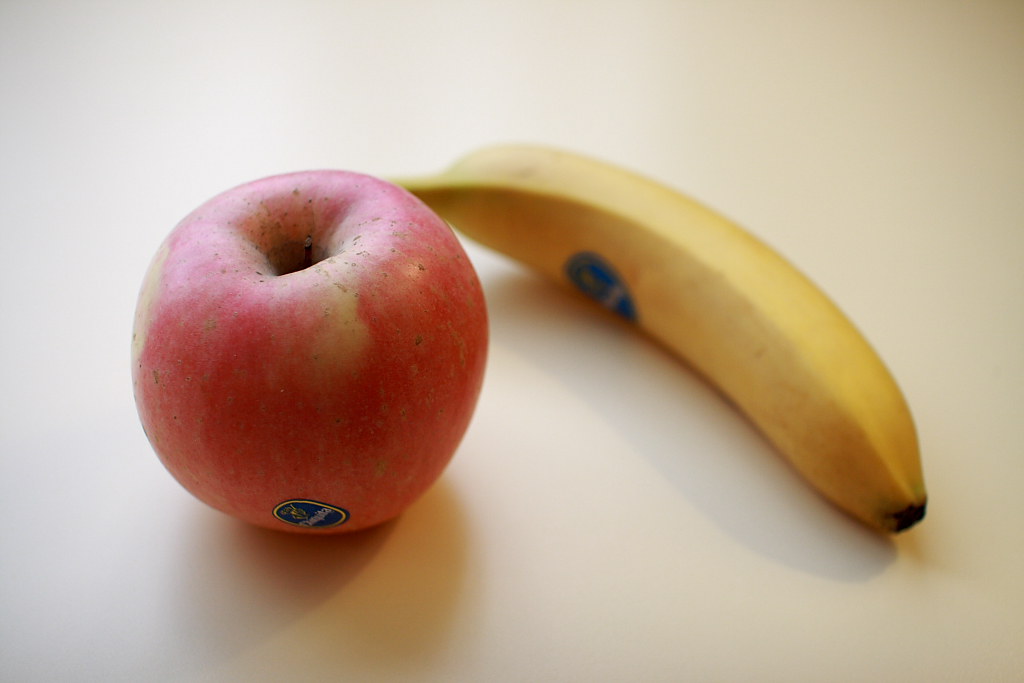In landscape orientation, the photograph captures two pieces of fruit on a light cream-colored surface that could be a table or floor. The left side of the image features a light gray background gradient, transitioning to a more yellow tone towards the right.

On the left side of the image, a red apple stands upright. The apple is ripe, with a brown stem situated at the top center and surrounded by a slightly darker indentation. The apple’s surface is marked with numerous small, light brown spots, particularly concentrated near the top. It has a yellowish tint on its left side and bears a Chiquita label at its bottom, indicating the brand.

To the right of the apple lies a perfectly ripe banana, positioned on its side. The banana’s stem is located behind the apple, pointing leftward, while the other end of the banana, which is dark black, points downward to the right. The banana also features a Chiquita label, situated on its left side.

Together, the apple and banana create a vivid and appealing still life composition, enhanced by the contrasting background and attention to detail in the fruits' textures and colors.